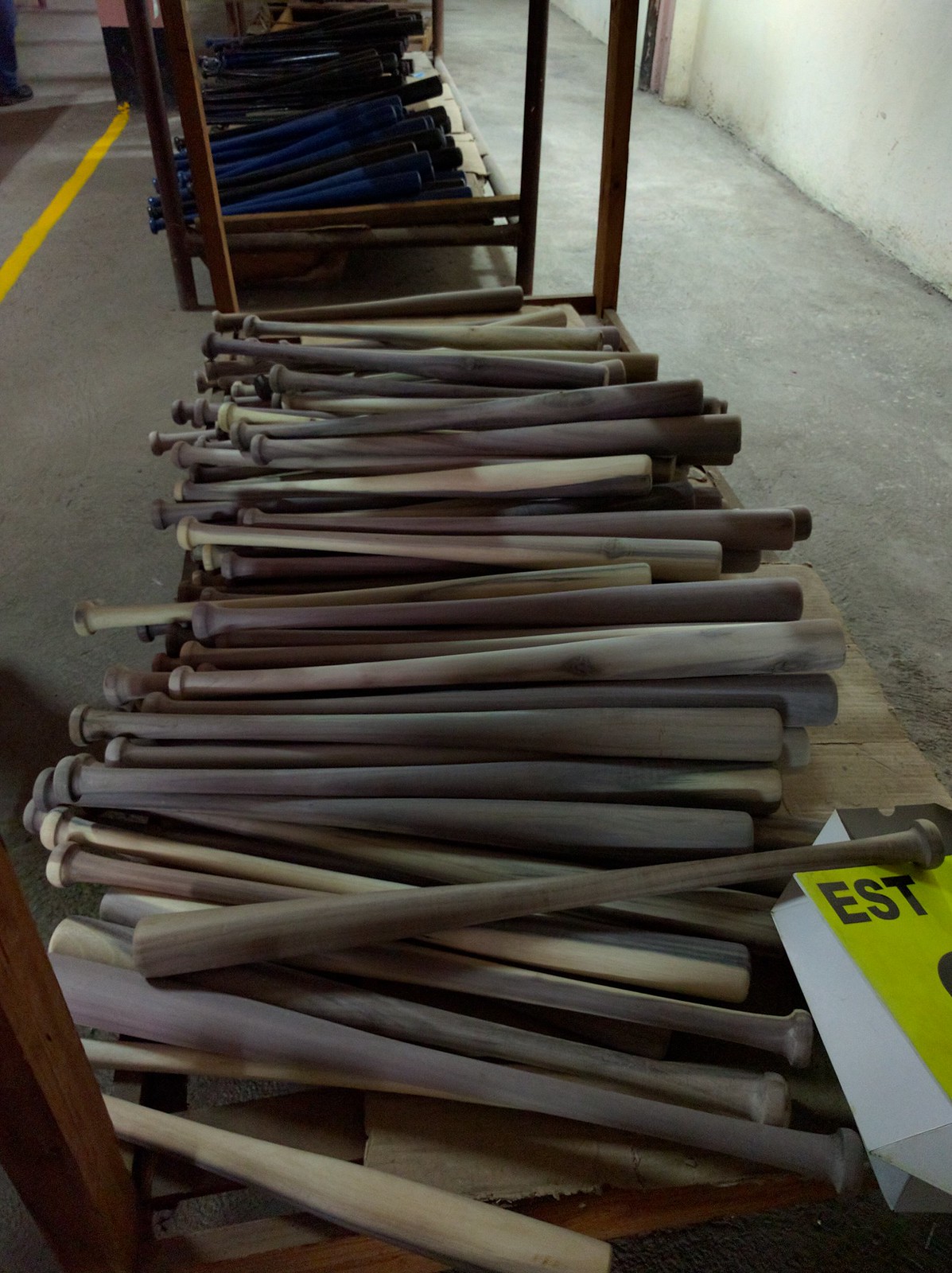The image depicts a plethora of wooden baseball bats in various colors, including light brown, grey, dark blue, and black, arranged meticulously within a warehouse. The bats are separated by color groups, with light brown and grey bats clustered together and the dark blue and black bats grouped separately. They rest on a low wooden shelf—there appears to be no shelf above it. Each shelf might hold between 50 to 100 bats. Within the scene, the warehouse has grey floors and walls, accented by a distinct yellow stripe running down the left side of the floor. In the lower right corner of the image, a piece of a yellow and white box is visible, bearing the black capital letters "EST." One bat notably angles above this box. Overall, the photograph captures the organized and industrial atmosphere of the storage space.